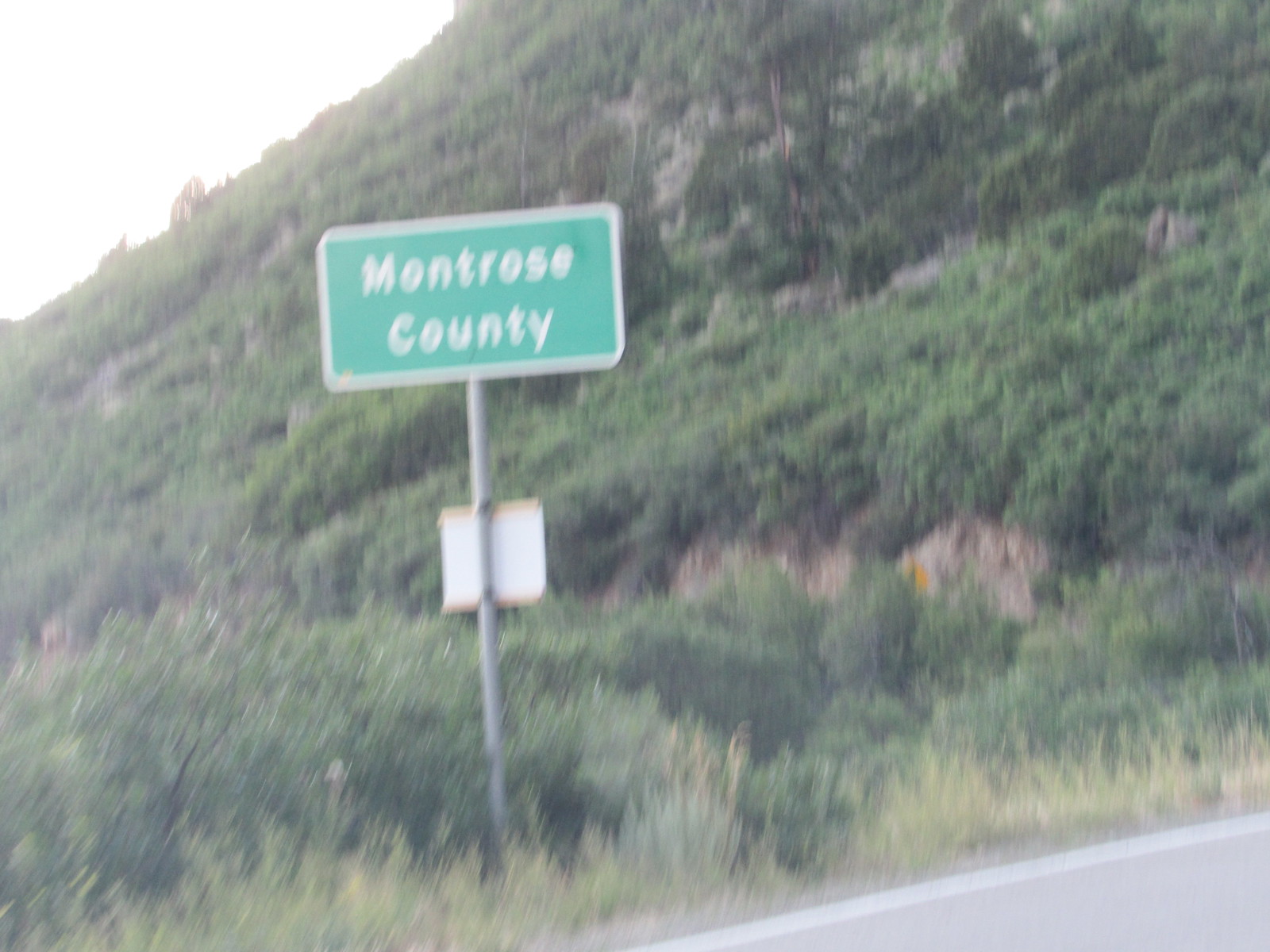A grainy, low-quality photograph captures a straightforward yet charming scene on a rural roadside. Dominating the foreground is a metal signpost, rising upwards and partially obscured by an indistinct attachment midway up, facing away from the camera. At the pinnacle of the post, a rectangular freeway sign with unrounded edges is prominently displayed. The sign, with its classic green background and clean white sans-serif text, reads "Montrose County" in title case. A neat white border frames the sign, enhancing its visibility.

The backdrop is a rugged mountainside, where rocky outcrops peek through a dense covering of vibrant green shrubbery. The road itself, an asphalt strip with a white edge line, is faintly visible and slightly blurred, complementing the overall texture of the image. No sidewalk is present; the scene is purely natural, with wild grasses and weeds flourishing by the roadside and around the signpost. The photograph is taken from an angle that slightly looks up towards the sign, adding depth to the composition.

To the top left, the setting sun casts a diffused, bright white light, suggesting either early evening or late afternoon. This subtle glow imbues the image with a warm, serene atmosphere, enhancing the sense of tranquility in this rural slice of Montrose County.